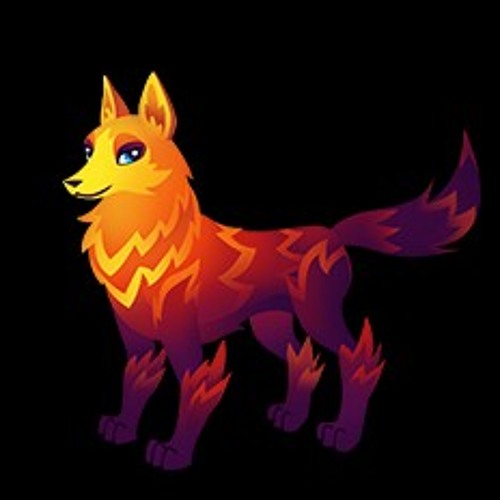This digital illustration depicts a vibrant, fox-like character set against a solid black background. The high-contrast backdrop makes the colorful and whimsical fox stand out prominently. The fox is adorned in a stunning ombre effect that transitions fluidly from yellow at its snout, through shades of orange and deeper red, and culminating in a striking purple hue. The creature's mesmerizing blue eyes and slight, knowing smile add a touch of personality. The top of its head starts in bright orange and yellow, resembling flickering flames, a motif echoed in the peaked, flame-like striping pattern throughout its fur. The fox's furry details are meticulously rendered, and its uplifted tail, bushy and vibrant, adds to the dynamic look. Although the image is slightly pixelated and maintains a cartoonish, animated quality, it brims with lively colors and intricate shading that give the character a captivating, almost fiery appearance.